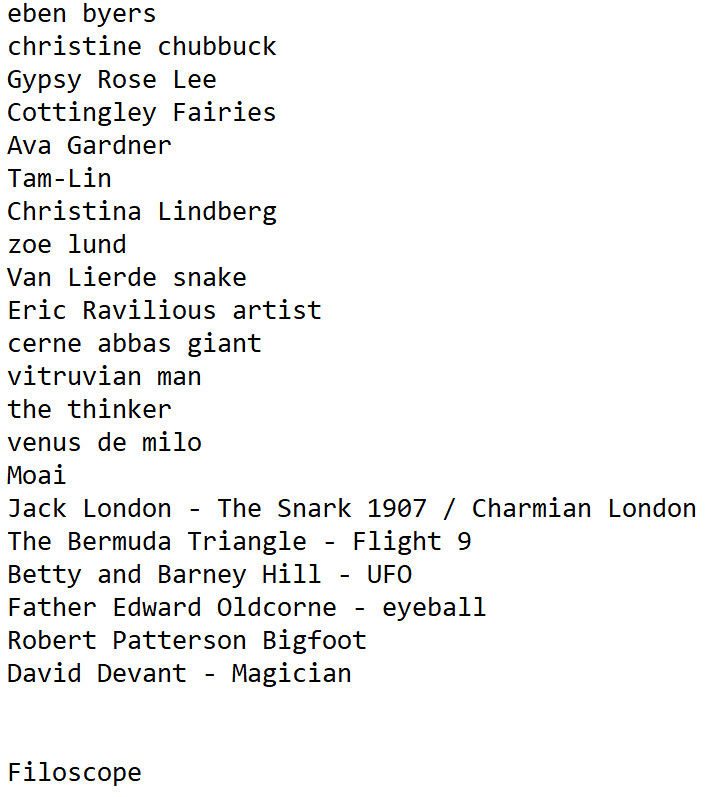The image features a typewritten list of names and terms in black font on a plain white background, all left-aligned in a vertical column. The text begins with "Eben Byers", followed by "Christine Chubbuck", "Gypsy Rose Lee", "Cottingley Fairy", "Ava Gardner", "Tam Lin", "Christina Lindberg", "Zoe Lund", "Van Leerdensnake", "Eric Ravilous Artist", "Cerne Abbas Giant", "Vitruvian Man", "The Thinker", "Venus De Milo", "Moai", "Jack London, The Snark 1907, Charmian London", "The Bermuda Triangle, 1889", "Betty and Barney Hill, UFO", "Father Edward Oldcorn, Eyeball", "Robert Patterson, Bigfoot", "David Devant, Magician", and concludes with "Philoscope".